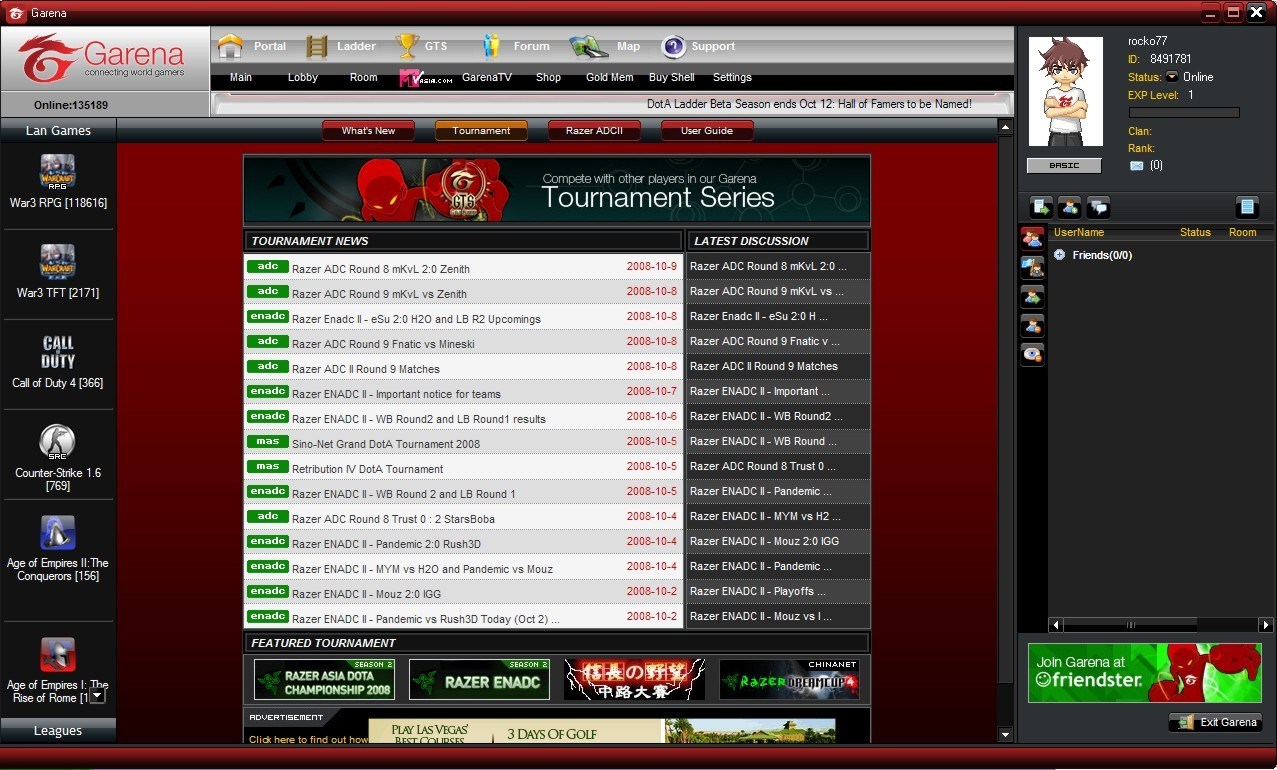**Caption:**

This is a screenshot of a nostalgic, old-school message board forum dedicated to video games, likely from Garena. The design harks back to early internet days, characterized by a solid top bar featuring the website name and a user profile section on the right side that displays information about friends and other user details. The low-quality screenshot further emphasizes its vintage nature, featuring pop-up ads and a simplified layout with prominent red and gray tones that starkly contrast with the web designs of 2024.

On the left side, there's a section labeled "LAN Games" listing various classic games such as Call of Duty 4, Counter-Strike 1.6, and Age of Empires 2, accompanied by small thumbnail images. The center of the screen highlights the forum's main content area, with a banner labeled "Tournament Series" displaying a red mascot figure believed to represent Garena. Below this banner, users can view tournament news and the latest discussions, identifiable by posts with dates from 2016 and 2018, adding to the retro feel of the site.

Further down, there's a section titled "Featured Tournament" showcasing images of various tournaments, though the details are hard to discern. Visible names include Razer and ADC, along with some Japanese text, alluding to the diverse gaming communities engaged on this platform. Overall, this screenshot captures the essence of an old-school gaming forum where enthusiasts could discuss and participate in gaming tournaments.